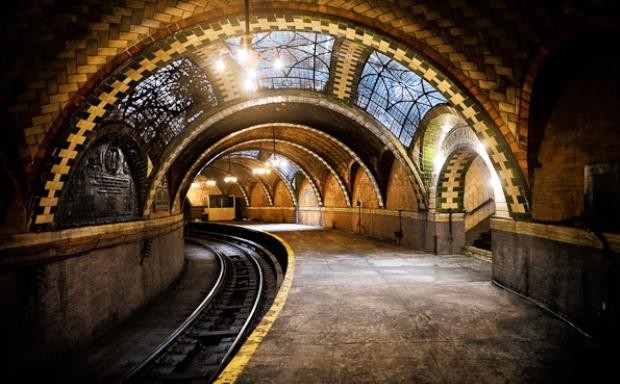This photograph captures a stunning underground tunnel designed for a train. The tunnel is adorned with ornate archways and ceiling decorations that feature crisscrossed stones of gold and red, forming a braided, U-shaped pattern. The highly decorated roof includes skylights with metal bars, allowing natural light to illuminate the intricately tiled interior. The tiles are shaped like bricks and contribute to the tunnel's rich hues of brown and black. In the center, a single curved train track runs alongside a golden guideline. The left side of the tunnel features a staircase descending into the scene, while chandeliers with multiple light bulbs hang in a straight line along the ceiling, adding to the tunnel's opulent atmosphere. Toward the back, a white square booth is visible, enhancing the detailed and lively underground environment.